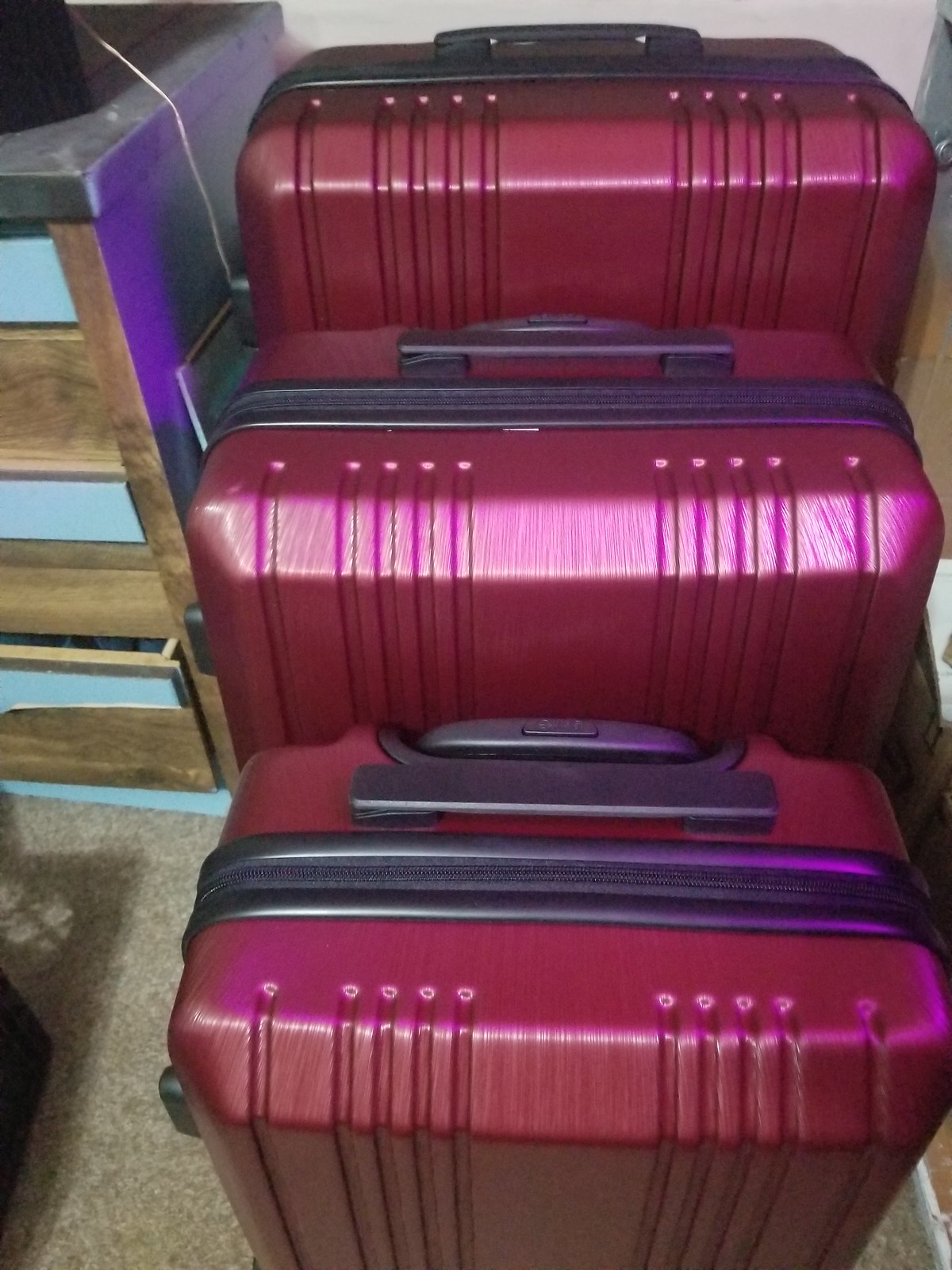This photograph depicts three hard-shell suitcases arranged in a stair-step formation, with the smallest in the front and the largest in the back. Each suitcase features a reddish-purplish color, transitioning from hot pink to burgundy, with black handles and zippers. The suitcases are part of the same set, characterized by engraved lines with distinct patterns – single lines, followed by groups of four lines. They are positioned on a beige speckled carpet beside a wooden piece of furniture that resembles a combination of an entertainment center and a filing cabinet, which has three drawers and a TV on top. The bottom drawer is slightly ajar, revealing a bit of its contents. The scene is set indoors, against white walls, under artificial lighting, which casts subtle reflections and shadows on the suitcases.